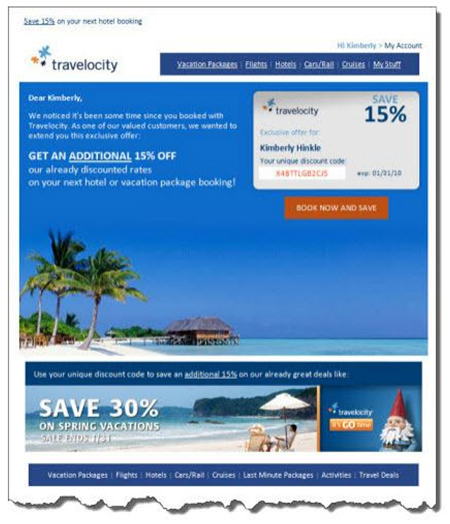The image is a promotional advertisement from Travelocity offering significant discounts on hotel bookings and vacation packages. In the top left corner, bold text announces, "Save 35% on your next hotel booking." The header also includes links to various categories such as vacation packages, flights, hotels, cars, cruises, and a section labeled "My Stuff." A greeting reads, "Hi, Kimberly," inviting her to view her account.

The main body of the advertisement begins with, "Dear Kimberly, we notice it's been some time since you've booked with Travelocity. As one of our valued customers, we wanted to extend to you this exclusive offer." Further down, a bold message states, "Get an additional 50% off already discounted rates on your next hotel or vacation package booking." The visual elements of the ad feature palm trees, a camera icon, and scenic images of blue waters and a white sandy beach on the left.

The top right corner prominently highlights an exclusive offer for Kimberly Hinkle, stating, "Save 50% exclusive offer for Kimberly Hinkle." The offer includes a discount code, emphasized in red letters, and an expiry date of "01.01.10." An orange rectangle button below urges, "Book now and save."

Near the bottom, the text advises, "Use your unique discount code to save an additional 50% on already great deals," mentioning a 30% discount on spring vacations and other packages. Below this, Travelocity's iconic gnome is displayed, with corresponding service categories listed: vacation packages, flights, hotels, cars/road travel, cruises, last minute packages, activities, and travel deals. The entire advertisement is designed to look like it’s on a piece of paper with frayed edges, adding a casual, friendly touch.